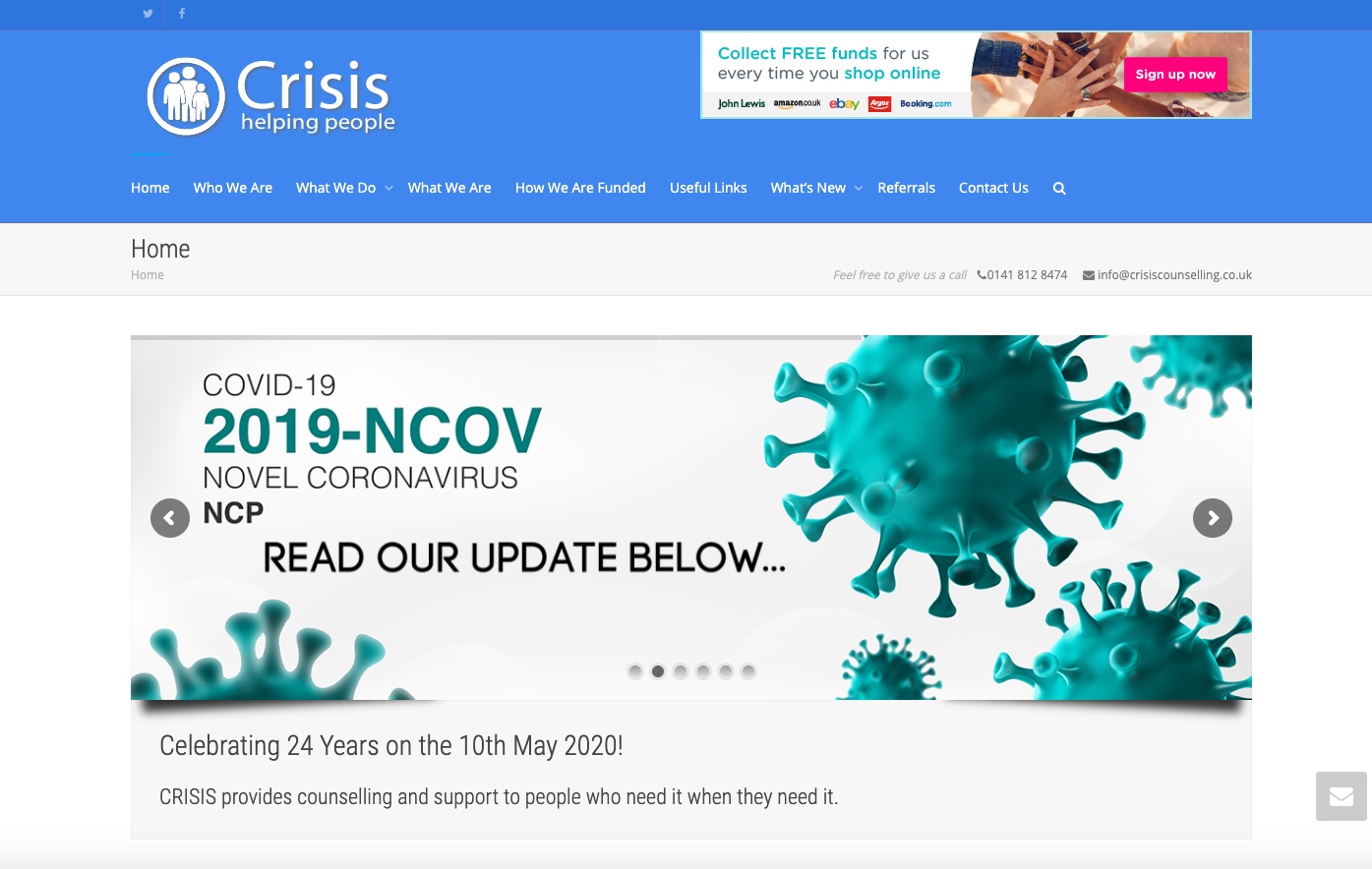An intricate, digitally-designed image displays various informative elements related to a crisis support organization. A large blue circle sits prominently in the center, adorned with icons for Twitter and Facebook. Three silhouetted figures, representing a family, are depicted within the circle, symbolizing unity and support. In a speech bubble, the name "Terai" is associated with a message urging viewers to "collect free funds for us every time you shop online. Sign up now."

The background features an array of phrases such as "Who we are," "What we do," "How we are funded," "Useful links," "What's new," "Referrals," and "Contact us," indicating the website's comprehensive resource sections. Floating nearby, COVID-19 related information appears, including terms like "19-NCOV," "normal coronavirus," and "NCP," suggesting important health updates.

Abstract elements, including blue, hollow, spirit-like figures traveling through a tunnel, hint at the viruses described in the text. An overlay commemorates "Celebrating 24 years on the 12th of May 2020," highlighting the organization's longevity and ongoing commitment. Below, a gray square, bordered with metallic elements, underscores the website’s structural segments. The predominant blue-themed design provides a sense of calm and trust, reinforcing the organization's mission to offer counseling and support during crises.